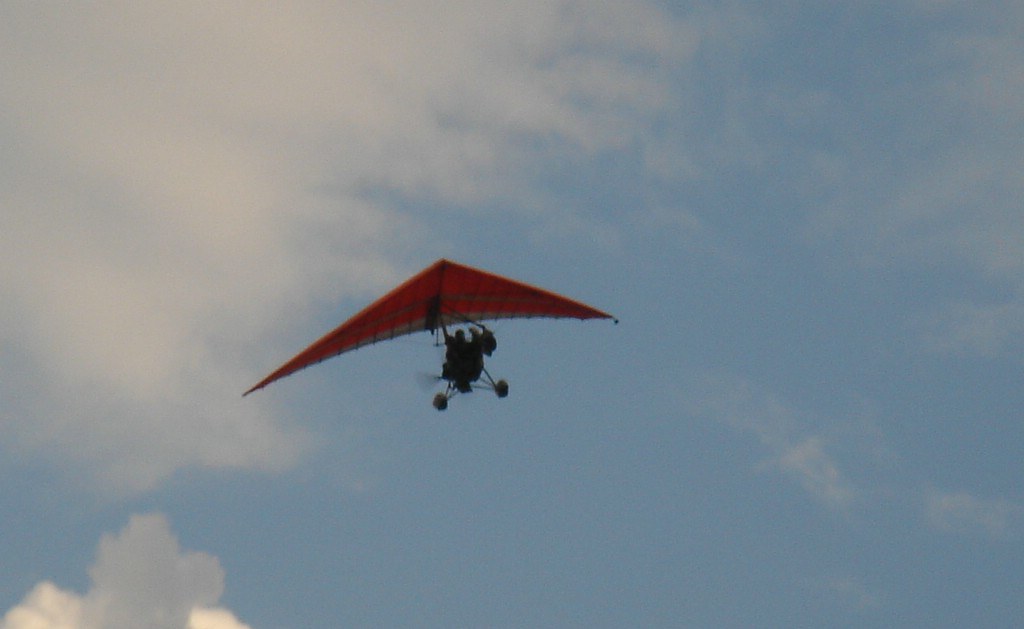The image captures an outdoor scene oriented towards the sky, likely taken close to sundown given the light blue tint and some darker hues in the sky, accompanied by fluffy white clouds primarily in the upper left. The focal point is a powered hang glider with an orange, triangular wing featuring white edges. Below the wing, a person is visible, seated within a mechanical frame, likely housing an engine and a spinning propeller. The glider is equipped with landing wheels and is connected to the hang glider by a pole. Due to the backlighting from the Sun, positioned behind and to the left, the person appears as a shadow against the sky, which further emphasizes the vibrant colors of the glider itself.